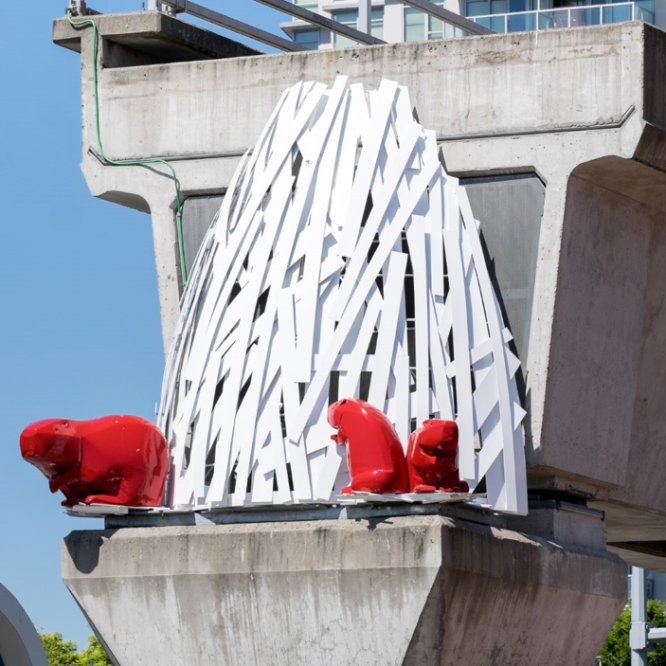The image captures an outdoor scene featuring a peculiar concrete structure, which appears to be some kind of abstract or artistic installation. The primary focus is a large, at least two or three-story concrete platform, slightly resembling an observation tower or a diving platform, though there is no water or diving board present. This white concrete structure is characterized by its surface stains and a partially obscured top.

At the base of this concrete platform, there is a cut white paper pyramid situated atop a platform. Beside it, there are three striking red statues of gopher-like animals, made from a glossy, almost porcelain-like material. One of these statues is leaning over and looking into the white pyramid, another is standing upright and looking towards the camera, while the third is facing left and positioned nearby.

The background features an observation deck or control room with glass walls and metal bars, potentially 40 feet in height, adding an industrial or futuristic element to the scene. The entire setting is illuminated by daylight, with a blue sky overhead and some trees visible at the bottom of the image. Overall, the combination of concrete structures, vivid red gopher statues, and the abstract paper pyramid creates a visually intriguing and surreal outdoor art scene.